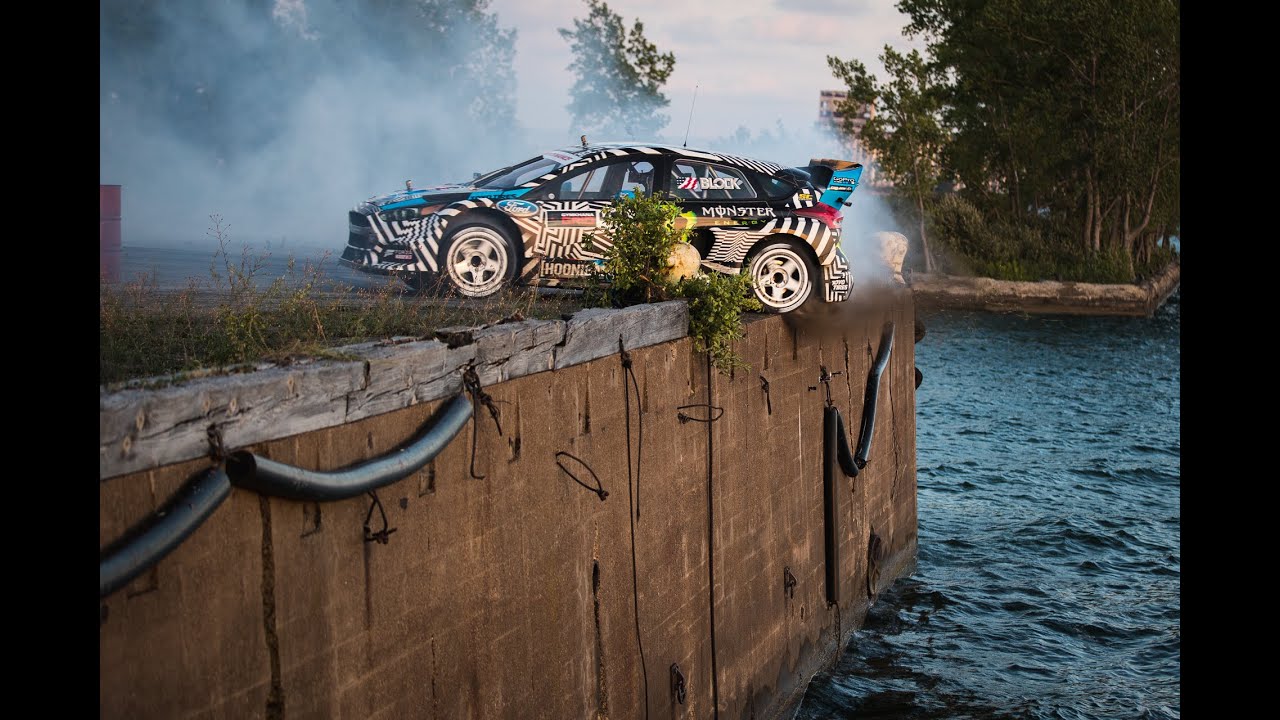In this striking photograph, a black and white zebra-striped rally car teeters precariously on the edge of a wooden pier. The rear left tire hangs over the dark blue water below, captured in the heart-pounding moment of either a daring escape or a close call. The car, adorned with intricate stripes and turquoise accents on the hood and rear spoiler, emits thick smoke from its spinning tires, creating a greyish haze in the atmosphere. Positioned centrally in the image, the car faces left while the viewer sees its dramatic side view, accentuated by text along the windshields and doors. The brown wooden pier, topped with a grey ledge and patchy green grass, stands high above the water, with tall green trees and a greyish sky forming the backdrop. The setting exudes a high-octane sports or automotive vibe, capturing the intensity and thrill of the moment.